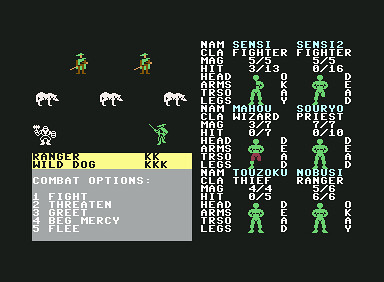Screenshot of an old-style 1980s RPG video game. The display is wider than it is tall, with a black background. On the right side, there's a table of information without borders, resembling a high score table. It features a series of abbreviations: N-A-M (name), C-L-A (class), M-A-G (magic), H-I-T (hit points), and lists parts of the body such as head, arms, torso, and legs. Green indicators show statuses like "okay" or "dead."

On the left side, there are icons representing characters and three gray wolves. A box in the lower left-hand corner displays terms like ranger, wild dog, and combat options, indicating the control panel for gameplay actions. This appears to be a classic RPG game from the 1980s.